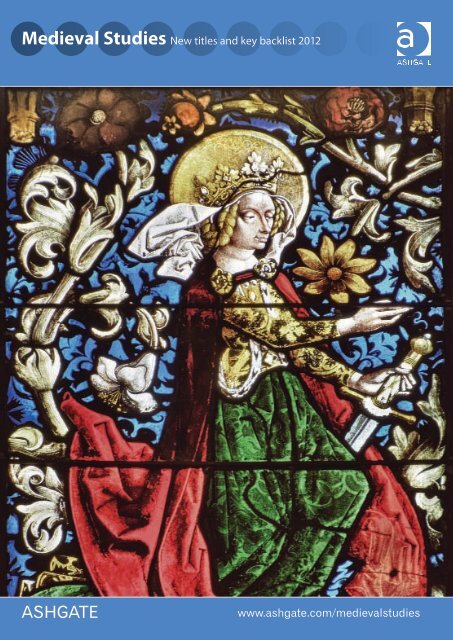The cover of the magazine "Medieval Studies: New Titles and Key Backlist 2012," published by Ashgate, features a striking artwork evocative of medieval times. The top and bottom sections of the cover display white text on a medium blue background, with a fading circle that runs through the words "Medieval Studies" to the right. The Ashgate logo, consisting of an off-center 'A' encircled in white with a blue background, is prominently featured.

Centrally, the cover showcases a detailed stained-glass depiction of a saint, identifiable by a gold halo against a blue, sky-like background. The saint wears a green robe with long gold flowery sleeves and a red cape draped to the ground. The figure is also adorned with other gold elements, suggesting a crown or some form of headpiece. Surrounding the saint are various pale cream and blue floral motifs, enhancing the medieval aesthetic.

This intricate artwork is complemented by the cover's text, which includes the title and the publication's details, emphasizing its focus on medieval studies and the key literature available from Ashgate in 2012.